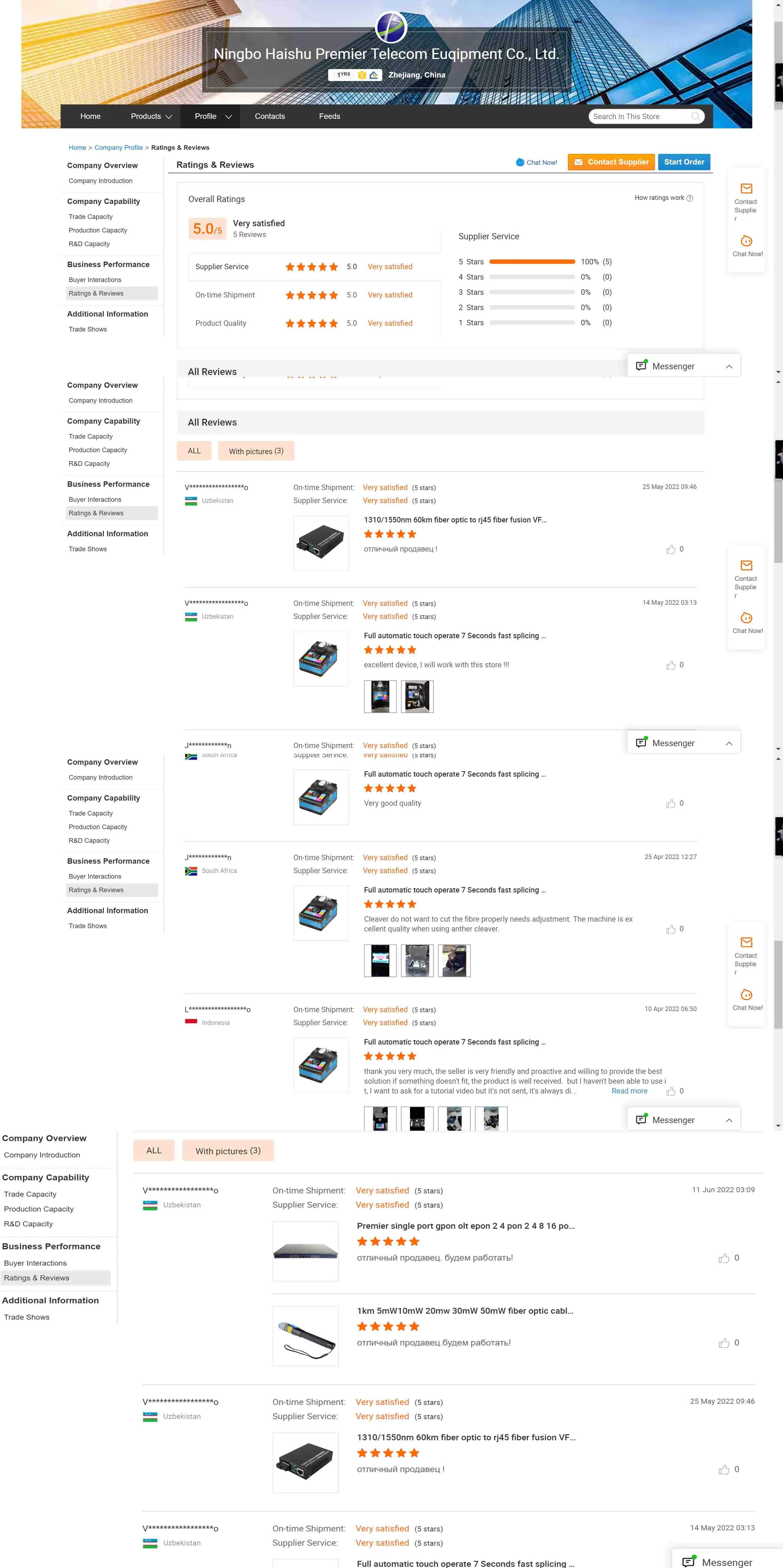The image depicts a text search bar on the website of Ningbo Heishu Premier Telecom Equipment Co. Ltd. Surrounding the search bar are multiple ratings and reviews evaluating the company's performance. The overall ratings are highly positive, with detailed metrics showing a perfect score of 5 out of 5 in several categories: supplier service, on-time shipment, and product quality. 

The first review, highlighted at the top, gives an overall rating of 5 out of 5 and is labeled as "Very Satisfied." This particular review, dated May 25, 2022, at 9:46 AM, is from a user in Uzbekistan who praises the timely arrival of a fiber optic box or cable. 

The page features a total of six reviews visible in the initial listing, with several more reviews appearing at the bottom, revealing consistently high satisfaction ratings. These additional reviews either stem from similar users or possibly the same company, all indicating high trust and satisfaction in the products offered by Ningbo Heishu Premier Telecom Equipment Co. Ltd. 

The company appears to specialize in a variety of telecom equipment, although the exact nature of each reviewed device isn't easily discernible from the available information.